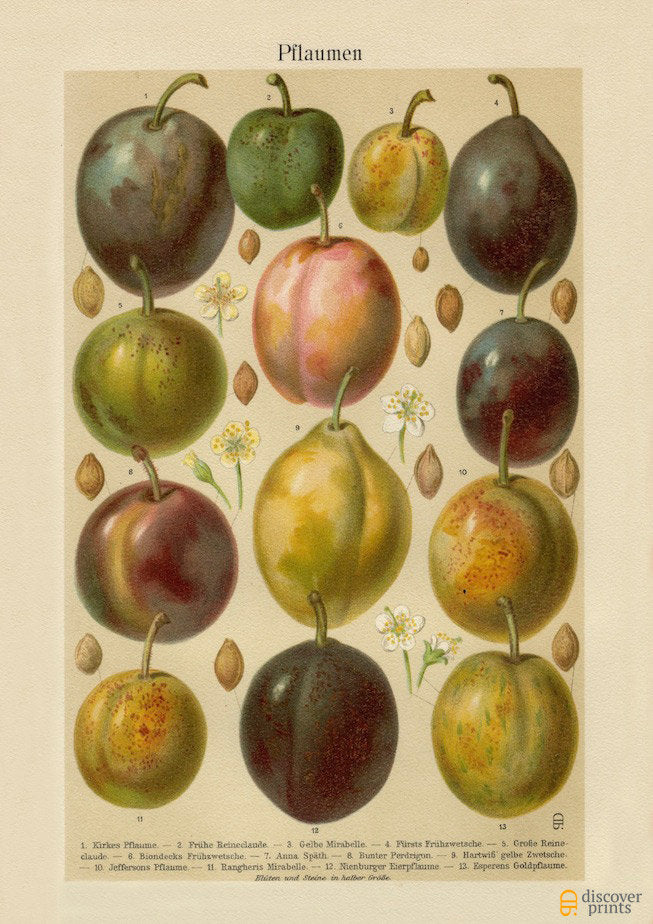This image is of a vertically aligned rectangular print with a light tan background. At the top, it features the word "Pflaumen" in a different language. The print displays thirteen various fruits, each rendered in a stylized, old-fashioned manner, resembling painted or drawn artwork rather than a photograph. The fruits, round or oval with stems, are arranged in four uneven rows: four on the top row, three in the second row, three in the third row, and three in the bottom row. Their colors range from red, yellow, and green to purple, black, gray, brown, and gold. Interspersed among the fruits are small squares resembling almonds and six floral illustrations with colors including white, yellow, and green, resembling daisies. The bottom part of the print contains text too fine to decipher, and the bottom right corner bears an orange logo with the words "Discover Prints" in gray.